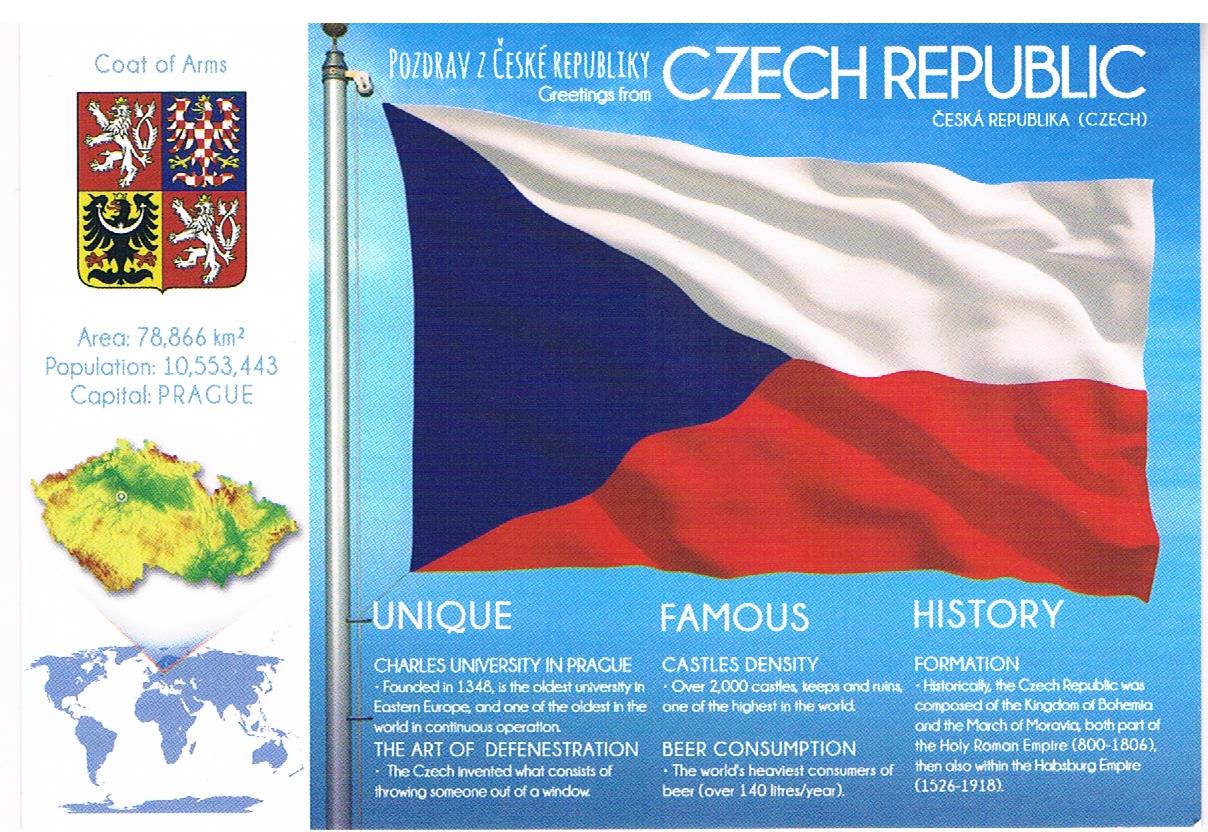This infographic about the Czech Republic features a vertical white column on the left and a blue background on the right. The left column showcases the country's coat of arms, which includes a lion on a red background in both the upper left and lower right quadrants, a black bird on a white background in the lower left quadrant, and a white and red Czech bird on a blue background in the upper right quadrant. Below the coat of arms, the infographic provides key statistics in blue lettering: an area of 78,866 km², a population of 10,553,443, and Prague as the capital. Beneath this, there are two maps - a topographic heat map of the Czech Republic colored green and yellow, and a world map indicating the country’s global location.

On the right side of the image, set against a blue background, the flag of the Czech Republic is prominently displayed in the upper middle. The flag features a blue triangle on the left, with white on the top right and red on the bottom right. Above the flag, the text reads "Greetings from Czech Republic" along with some words in Czech. Below the flag, three sections provide detailed information about the country under the headings "Unique", "Famous", and "History":

- **Unique**: Charles University in Prague, founded in 1348, is highlighted as the oldest university in Eastern Europe and one of the oldest in the world in continuous operation. It also mentions the Czech innovation of the art of defenestration, or the act of throwing someone out of a window.
- **Famous**: Notably, the Czech Republic boasts one of the highest densities of castles, with over 2,000 castles, keeps, and ruins. The country also has the world's highest beer consumption, with over 140 liters per person annually.
- **History**: The historical formation of the Czech Republic is detailed starting from its composition as the Kingdom of Bohemia and March of Moravia under the Holy Roman Empire from 800 to 1806, extending through its inclusion in the Habsburg Empire between 1526 and 1918.

Overall, the infographic provides a comprehensive visual and informative overview of the Czech Republic's key geographic, demographic, cultural, and historical facts.